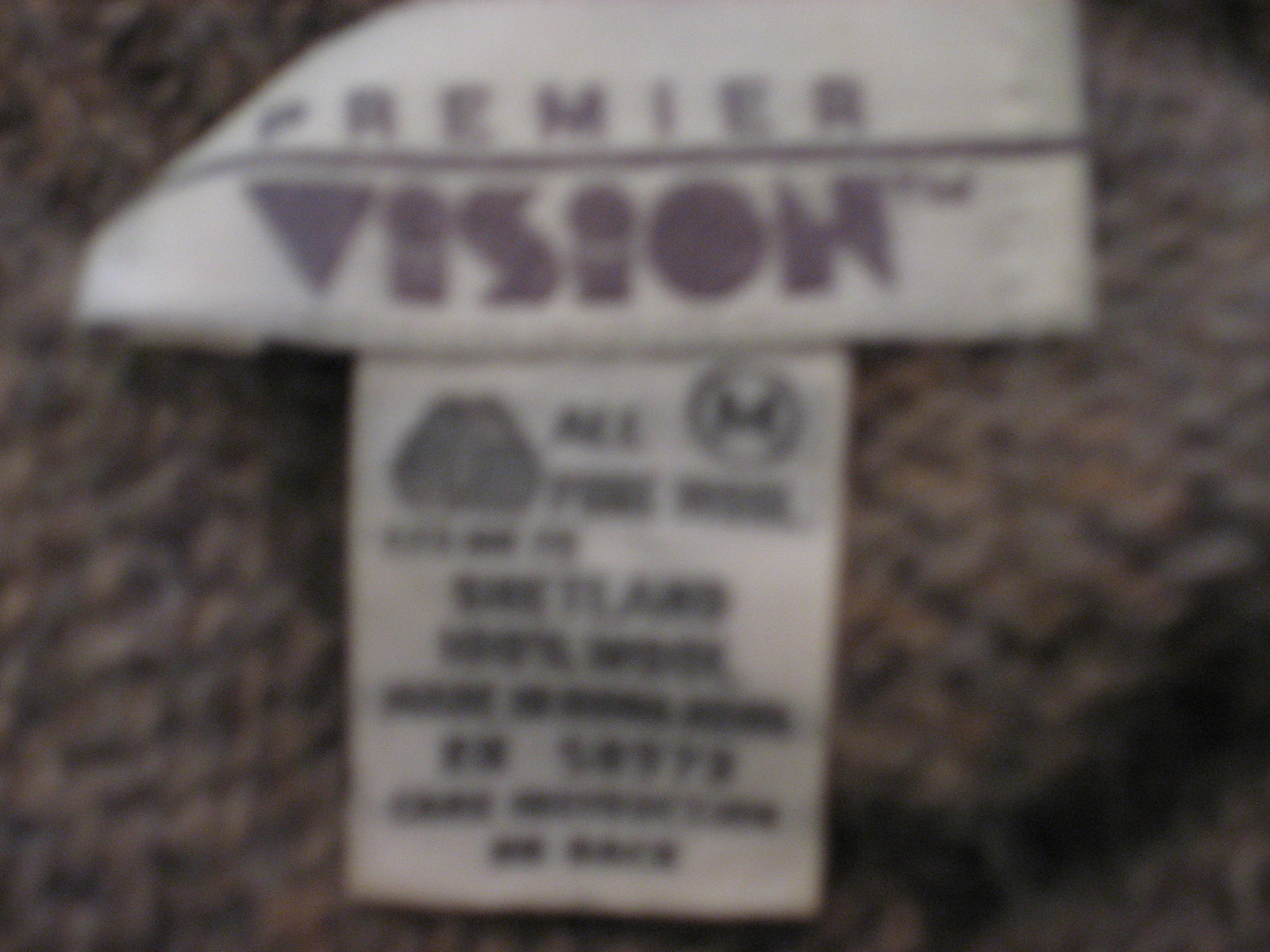This photograph showcases a close-up of a clothing label, though the image quality is notably blurry. The label is affixed to the inner lining of a garment crafted from a warm, woolly fabric characterized by various shades of brown. The primary label bears the name "Premier Vision" in deep purple text set against a white backdrop. Just beneath it, a secondary label details care instructions, presented in black text on a white background. However, due to the image’s lack of clarity, the care instructions remain unreadable.